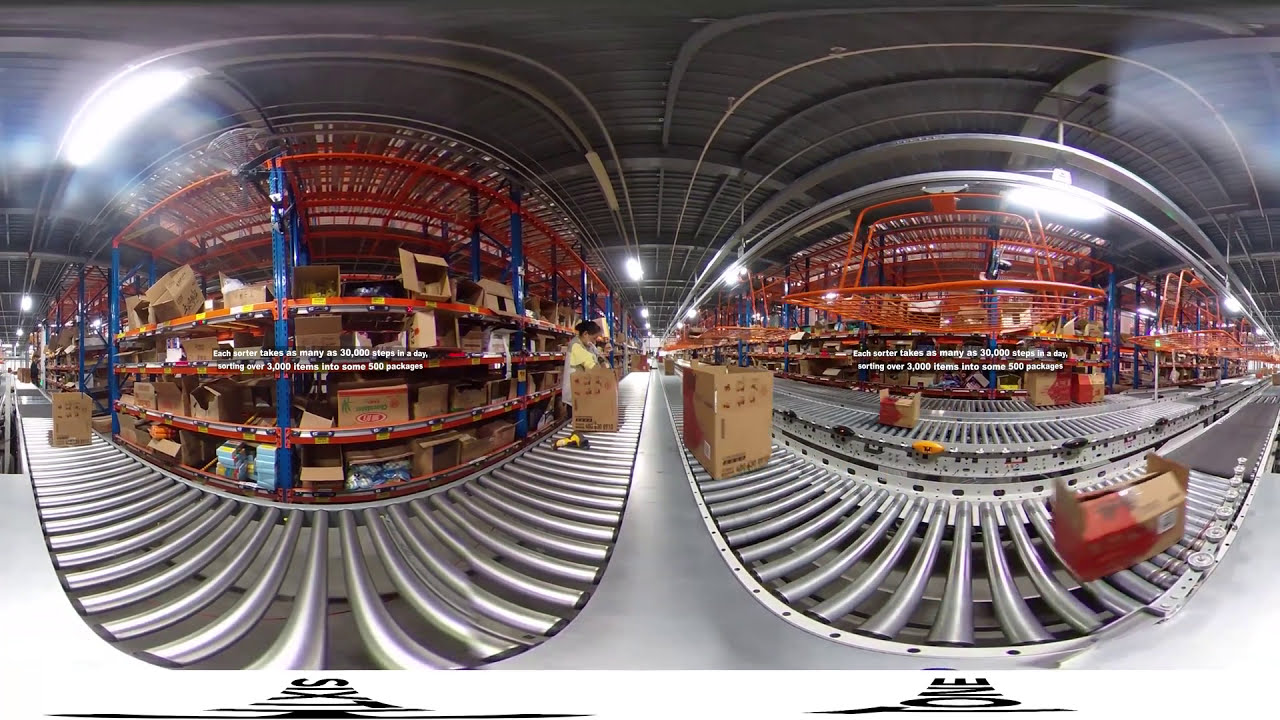This dynamic image, captured with a 360-degree panoramic fisheye lens, showcases a bustling warehouse featuring a central conveyor belt system. It's divided into two sections that appear slightly distorted due to the lens effect. In the center of the image, white text reads: "Each sorter takes as many as 30,000 steps a day, sorting over 3,000 items into some 560 packages," highlighting the efficiency of the workers. The conveyor belt extends the entire length of the warehouse, transporting open-top boxes towards workers positioned to the left. These workers are actively sorting and placing items into the boxes, amidst a backdrop of tall shelving units. The shelves, supported by orange and blue frames, stretch far into the distance and are densely packed with various items, predominantly brown boxes. The image vividly captures the fast-paced environment of an active supply line, reflecting the high level of productivity in this warehouse setting.